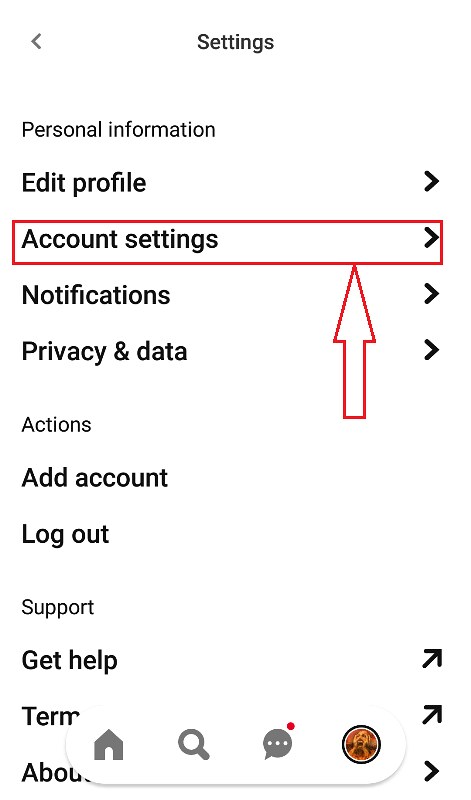This is a full-color screenshot depicting the settings menu of an application. The layout features a clean, white background with various sections and options organized neatly on the screen. At the top center, the title "Settings" is displayed prominently. Below are several main menu items arranged in a list format: "Personal Information," "Edit Profile," each with a right-facing caret indicating further options.

The next section is labeled "Account Settings" and includes options such as "Notifications," "Privacy and Data." This section is highlighted with a red rectangle, and a large red outlined arrow points upwards towards "Account Settings," emphasizing its importance.

Following this, the "Actions" section presents options for "Add Account" and "Log Out." Beneath this, the "Support" section offers "Get Help," "Terms," and "About."

At the very bottom of the screen is a navigational toolbar featuring a series of icons from left to right: a grayed-out home button, a search button, and a grayed-out message button adorned with a red notification dot. On the far right, there's the user’s profile picture encased in a circle.

Overall, the screenshot provides a comprehensive view of the application's settings interface, marked by intuitive organization and clear visual cues.